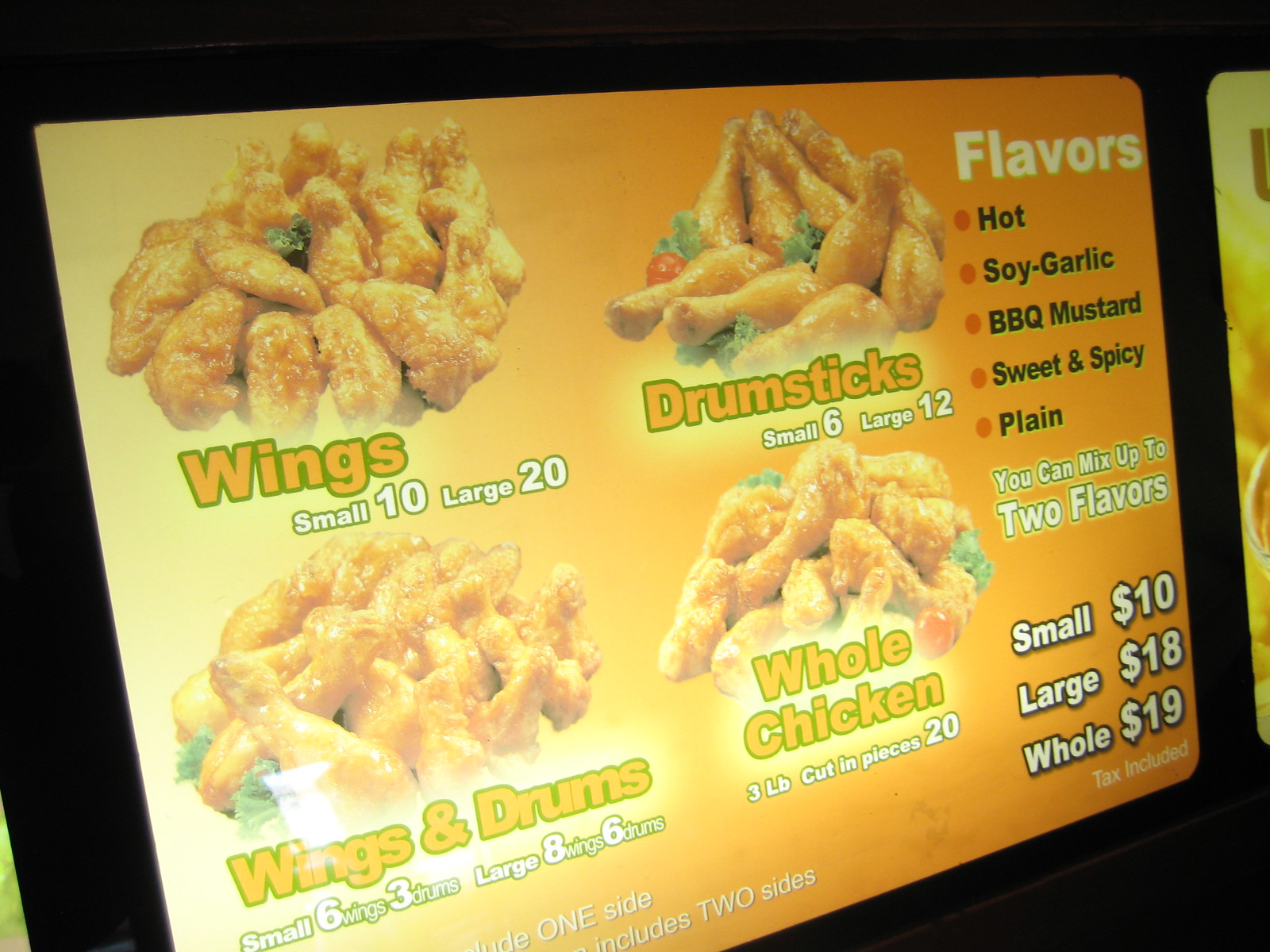This is an indoor color photograph of a brightly lit section of a restaurant menu sign, likely positioned above the cash registers in a fast-food establishment. The menu display is predominantly orange and yellow, featuring images of various fried chicken options arranged in a rectangular layout divided into four sections. 

In the upper-left section, there's an image of golden, sauced wings with text indicating "Wings," priced at Small $10, Large $20. Next to it, on the upper-right, is an image of similarly sauced drumsticks labeled "Drumsticks," with prices Small $6, Large $12. 

Below these, the lower-left section displays a combination platter labeled "Wings and Drums," detailing Small 6 wings and 3 drums, Large 8 wings and 6 drums. The lower-right section illustrates "Whole Chicken," describing it as a 3-pound chicken cut into 20 pieces.

On the right side of the display, under the header "Flavors" written in white text with bullet points, the flavors listed are Hot, Soy Garlic, Barbecue Mustard, Sweet and Spicy, and Plain. Additionally, it mentions that you can mix up to two flavors. Beneath this, the prices for the chicken sizes are reiterated as Small $10, Large $18, Whole $19. The overall background of the display is a vivid orange with a black border, giving it a striking and appetizing appearance.